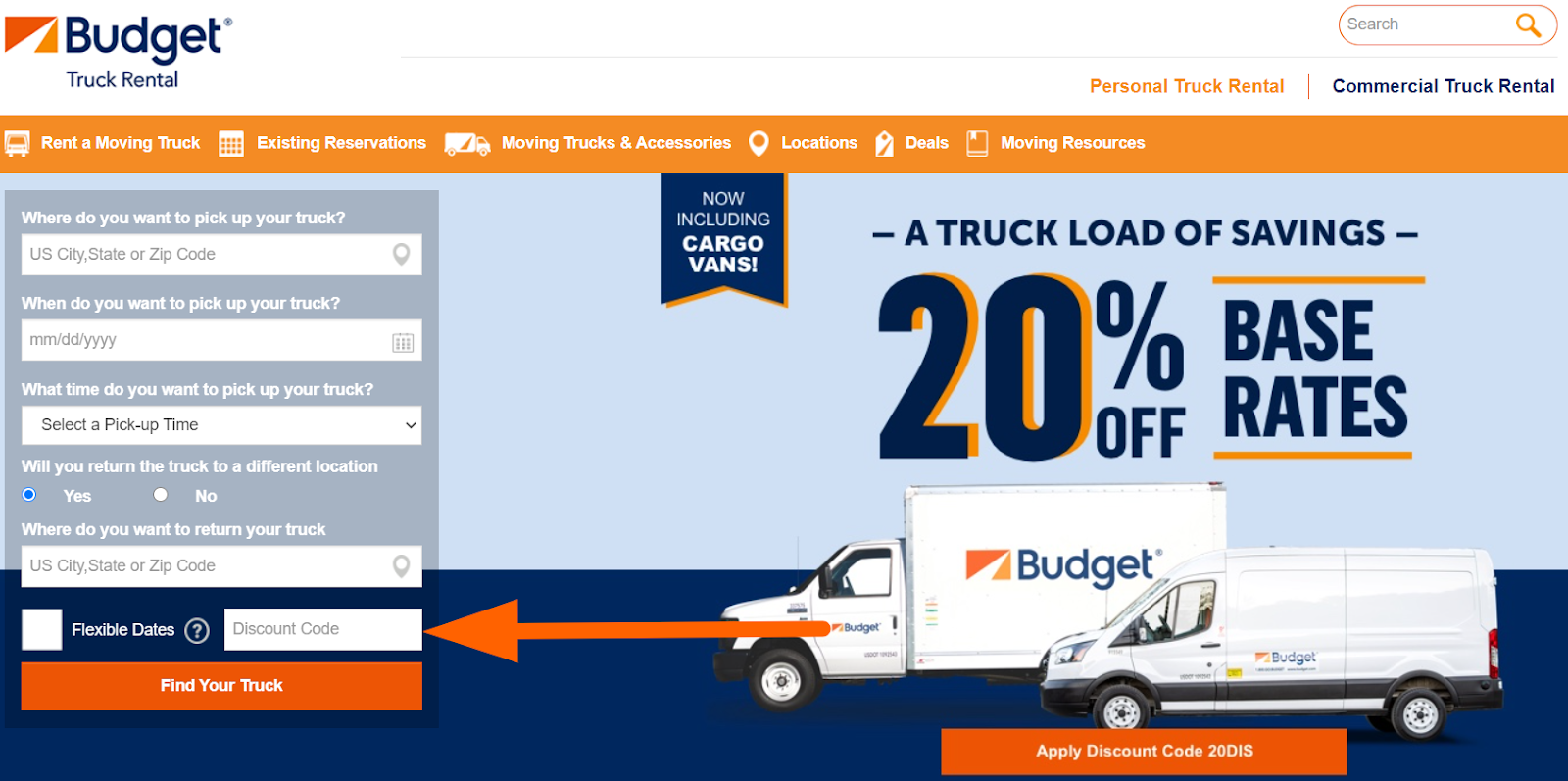This digital advertisement for Budget Truck Rental prominently features key details in a structured layout. In the top left corner, "Budget Truck Rental" is clearly stated beside an orange square. To the right, a search bar with a magnifying glass icon allows users to begin their search, with "Personal Truck Rental" in orange text and "Commercial Truck Rental" in blue text displayed nearby.

Users are prompted with various options for truck reservation: "Where do you want to pick up your truck?", "When do you want to pick up your truck?", "What time do you want to pick up your truck?", "Will you return the truck to a different location?" with a simple yes or no option, and "Where do you want to return your truck?" followed by a field to enter the return location.

The center of the advertisement showcases an illustration of a Budget rental truck and a Budget rental van, emphasizing the available vehicle options. An orange arrow points left towards an area where users can input a discount code.

Towards the bottom, a prominent orange rectangle with the text "Find Your Truck" serves as a call-to-action button. An informational section states "Now including cargo vans" in orange text, and an additional orange rectangle suggests applying the discount code "20DIS" for savings.

Overall, the advertisement provides a clear, user-friendly interface to assist customers in renting trucks, accompanied by offers and options tailored to their needs.